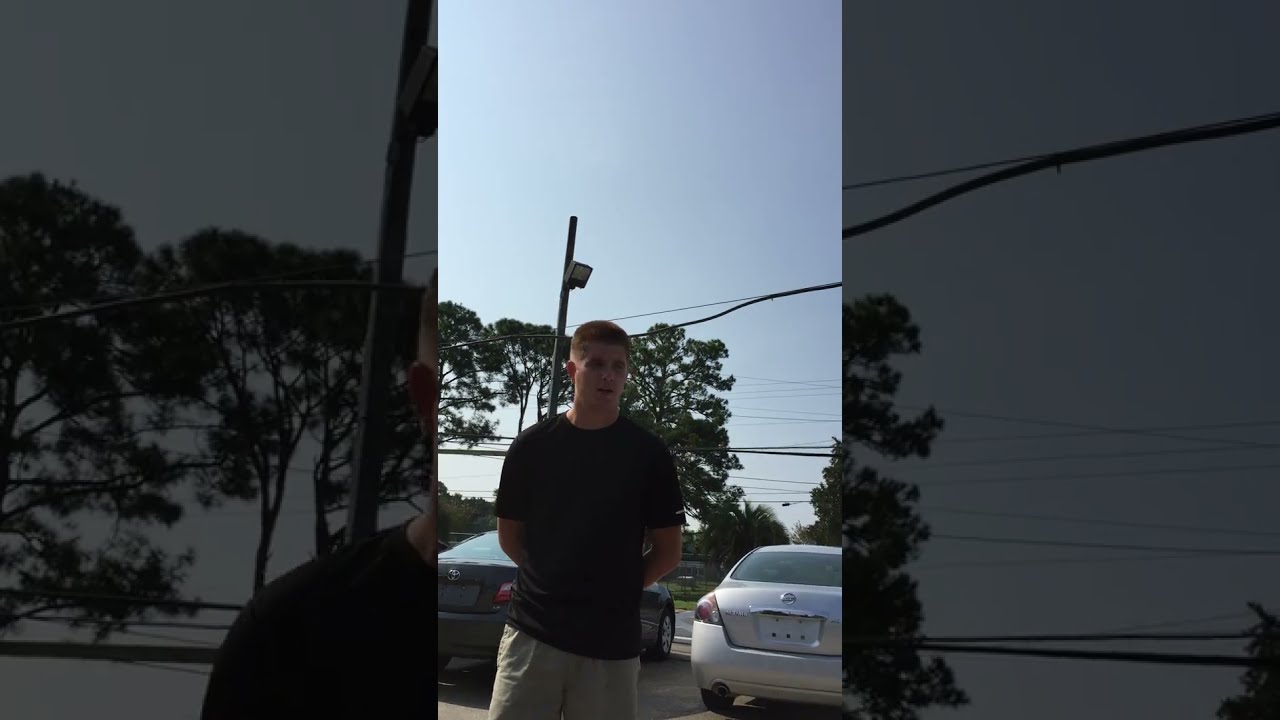In the center of the image, a young man, appearing to be in his late teens or early 20s, stands in a parking lot. He is wearing a black short-sleeved t-shirt and tan or khaki-colored pants with his hands behind his back. The man has short-cropped, reddish-brown hair, and is gazing off to his right. The image is framed with a thick black border on both the left and right sides, occupying about 70% of the total width. Behind him, there are two cars: a dark gray car on the left and a silver-colored car on the right, both missing their license plates. The parking lot is bordered by a dark asphalt road marked with white lines. A metal pole with a street light and multiple black wires extending in various directions stands nearby. On the opposite side of the road, a green area is fenced off with a black chain-link fence, and several green-leaved trees are visible. The sky above is completely clear, without any clouds.